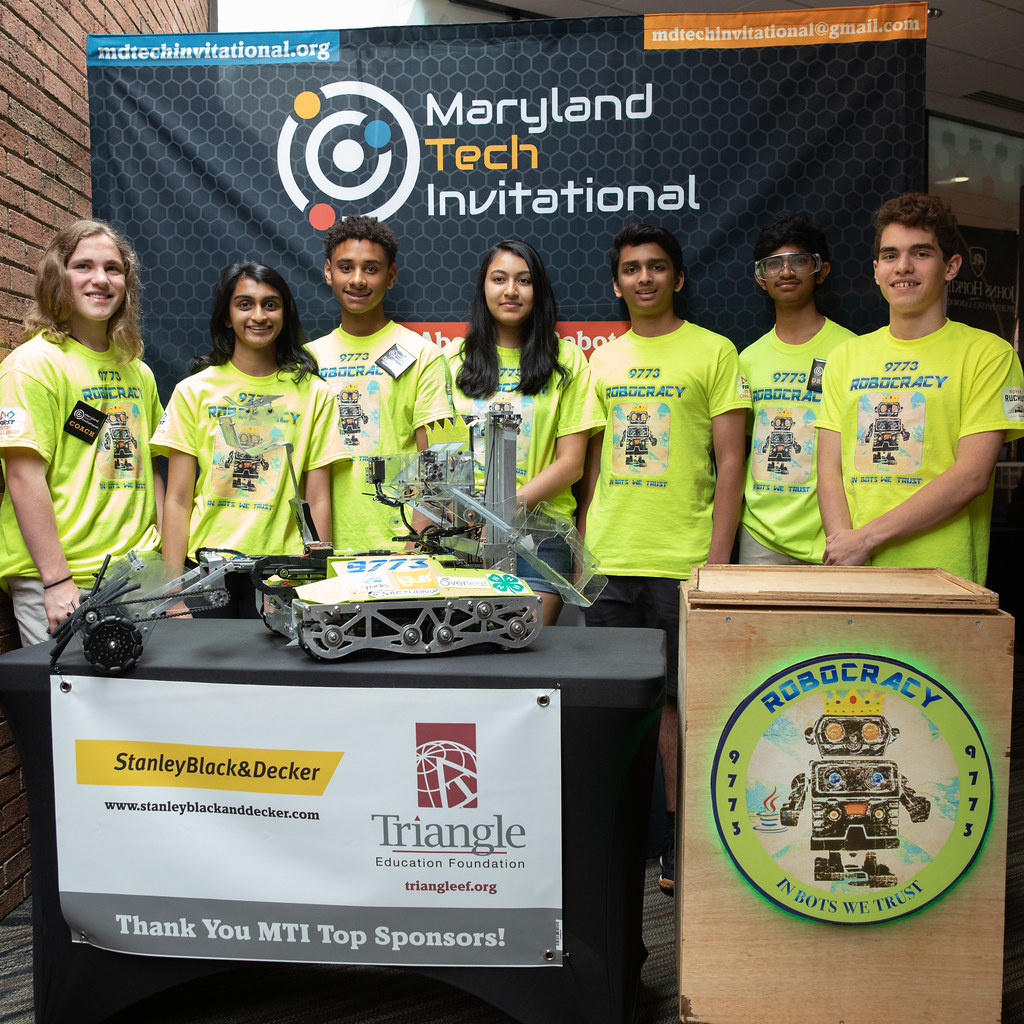A group of seven teenagers stands proudly in front of a gray sign adorned with a white, yellow, and blue logo that reads "Maryland Tech Invitational." Each member of the group wears a lime greenish-yellow shirt with the team name "9773 Robot Robocracy" and a picture of a robot. Their shirts also feature the tagline, "In bots we trust," and each teen sports a name tag. They are gathered behind a black-covered table that displays a robot vehicle with tread wheels, movable arms, and various plastic components. The table is decorated with a banner thanking top sponsors such as Stanley Black & Decker and the Triangle Education Foundation. To the right of the table, there is a podium with a sign that also bears the team's name and tagline. The scene suggests that these young participants are competing in a robotics competition at the Maryland Tech Invitational.